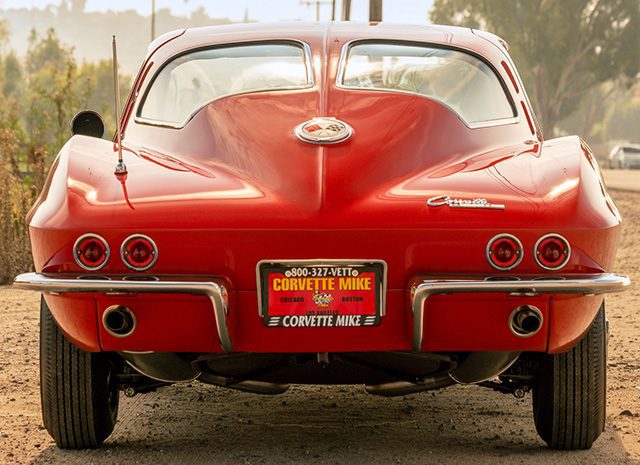This photorealistic image, which also has a computer-generated feel, captures the rear view of a pristine, red, older-model Corvette. The car's distinctive back windshield is split into two separate windows, one on the left and one on the right. It showcases silver, wing-like accents beneath each of the two pairs of headlights on the bumper. The focal point is the red license plate that reads "Corvette Mike" with the border displaying the number "800-327-VETT." The shiny vehicle stands out as it is parked on a dirt road, with small trees framing both sides of the scene, hinting at a sunny day. In the background, to the right, a small gray car is visible, adding depth to the otherwise dry landscape.